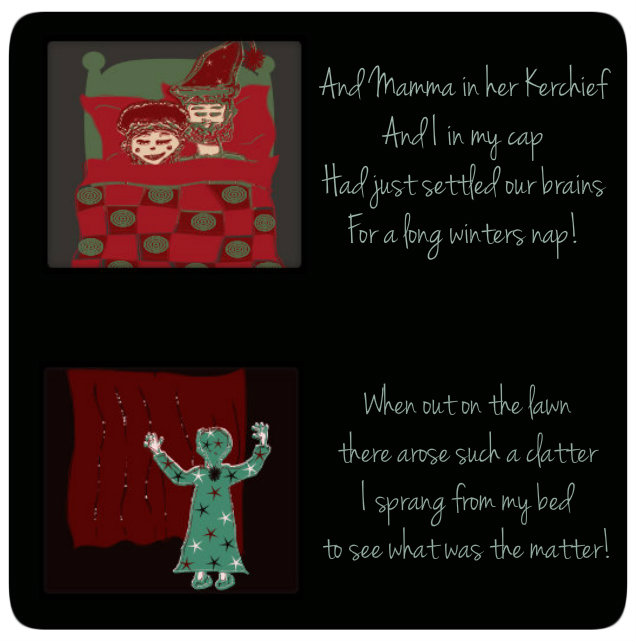This image, appearing to be a page from a book or a card, features a black background with white text on the right-hand side. The text reads, "And Mama in her kerchief and I in my cap had just settled our brains for a long winter's nap. When out on the lawn there arose such a clatter, I sprang from my bed to see what was the matter."

On the left side of the page, there are two illustrations. The top illustration depicts a man and a woman lying in bed. The man, sporting a big beard and a nightcap resembling a Santa Claus hat with a round ball at the end, wears a green bed shirt. The woman, with red cheeks and her hair tucked into a white nightcap, rests beside him. They sleep on a bed that has a green headboard and a red and green checkered bedspread.

Below this, the second illustration has a brownish background with red curtains blowing. In front of the curtains stands a small figure clad in a nightgown and slippers, waving both arms energetically. The details in both images accentuate a cozy winter bedtime scene, setting a tranquil yet whimsical mood.